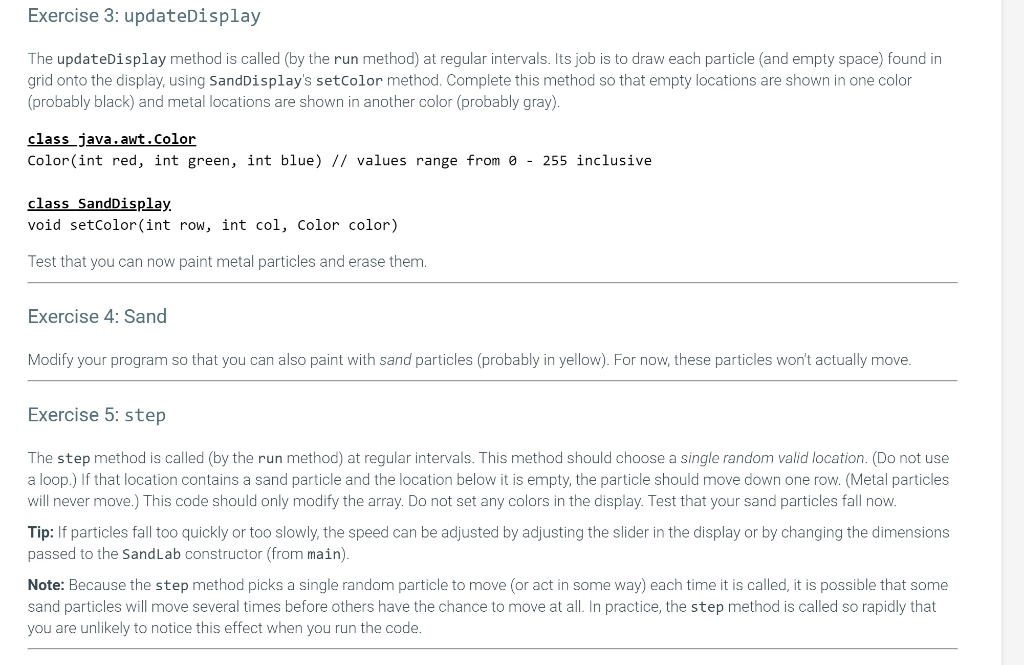**Detailed Caption:**

This image is a screenshot of a website, featuring text content related to a programming exercise. In the upper left-hand corner, the heading "Exercise 3: Update Display" is prominently displayed, with a capital 'D' on "Display." Directly below this heading is a detailed paragraph explaining that the "updateDisplay" method is invoked by the "run" method at regular intervals. Its purpose is to render each particle and the empty spaces within a grid onto the display, utilizing the "sendDisplay.setColor" method. The task entails completing the method such that empty locations are shown in black, while middle locations are depicted in gray.

Following the paragraph is a section of code references, starting with "class java.awt.Color," then "class SandDisplay." Below the code references, there's an instructional line indicating that users should now be able to paint metal particles and erase them.

Subsequent to this, the document transitions into "Exercise 4: Sand," which instructs users to modify their program to enable painting sand particles, presumably in yellow, though these particles will not move for now.

Lastly, "Exercise 5: Step" is introduced. This exercise requires the development of a "step" method that is called by the "run" method at regular intervals. The method's function should be to select a single random valid location.